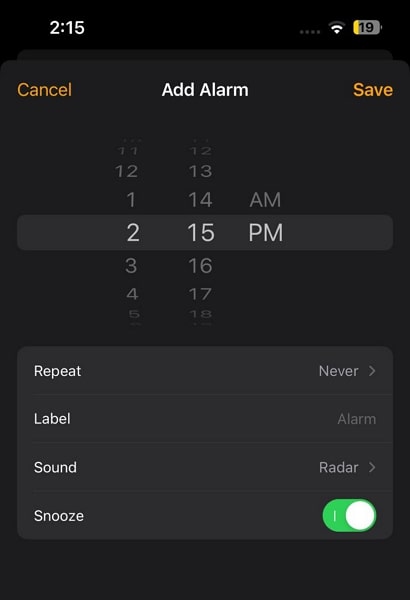This screenshot depicts the "Add Alarm" settings screen on a mobile phone with a black background. In the top left corner, the time is displayed as 2:15. Over in the top right corner, the battery level is shown at 19%. Moving to the middle top section, the screen title "Add Alarm" is prominently featured. Flanking this title, "Cancel" is written in orange on the left, and "Save" is on the right.

At the center of the screen, a digital time dial is set to 2:15 PM, allowing users to adjust the alarm time. Below the time dial, there are four rows of additional settings.

1. **Repeat:** The word "Repeat" is followed by a considerable space, then "Never" is displayed, indicating that the alarm is not set to repeat.
2. **Label:** Similarly, after a large space following the word "Label," the text "Alarm" appears, denoting the alarm’s label.
3. **Sound:** The word "Sound" is succeeded by a space, then by "Radar," indicating the chosen alarm sound.
4. **Snooze:** Finally, "Snooze" is written with a green toggled button next to it, signifying that the snooze function is enabled.

Each of these rows provides a clear and organized layout of settings, enabling users to easily customize their alarm preferences.